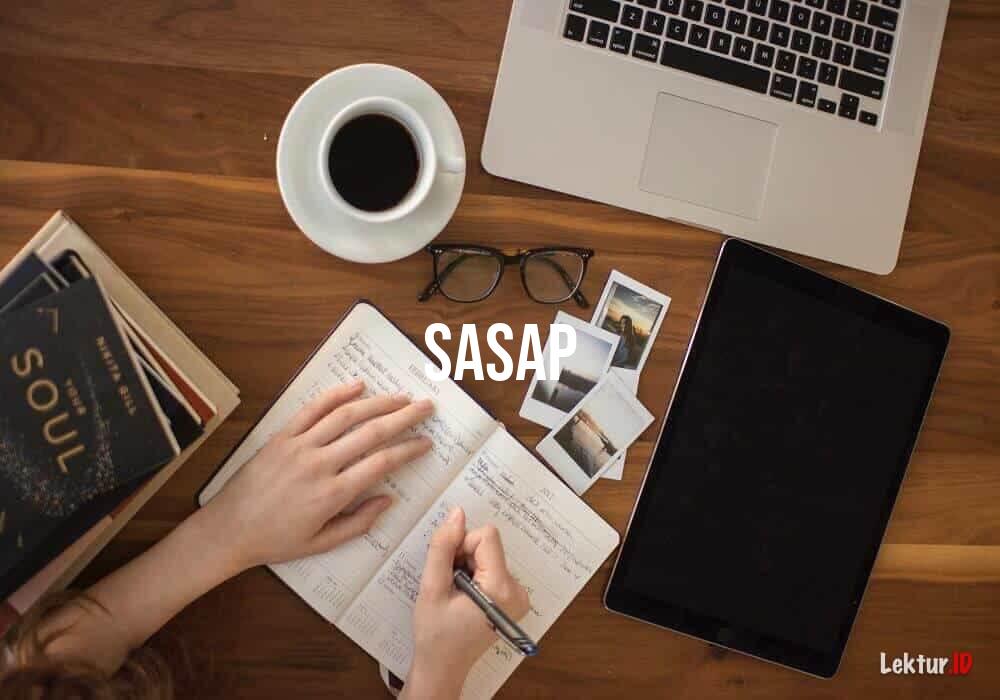This color photograph is captured in landscape orientation from a top-down perspective, showcasing a neatly arranged wooden table with a light reddish-brown hue distinctively displaying its woodgrain lines. Positioned at the top right of the image is a silver laptop with black keys and white lettering next to a white coffee cup on a matching saucer, filled with dark coffee. In the bottom left corner, there are five books stacked, with the topmost book titled "Your Soul." Adjacent to the books are a pair of brown eyeglasses, several printed photographs, and a black tablet with a blank screen. Central to the image is an open journal into which the right hand of a person, emerging from the bottom left, is writing with a pen, while their left hand assists. Overlaying the middle portion of the image is the text "S-A-S-A-P" in bold white letters. Finally, the bottom right corner features a small logo that reads "Lecture ID, L-E-K-T-U-R dot 10."